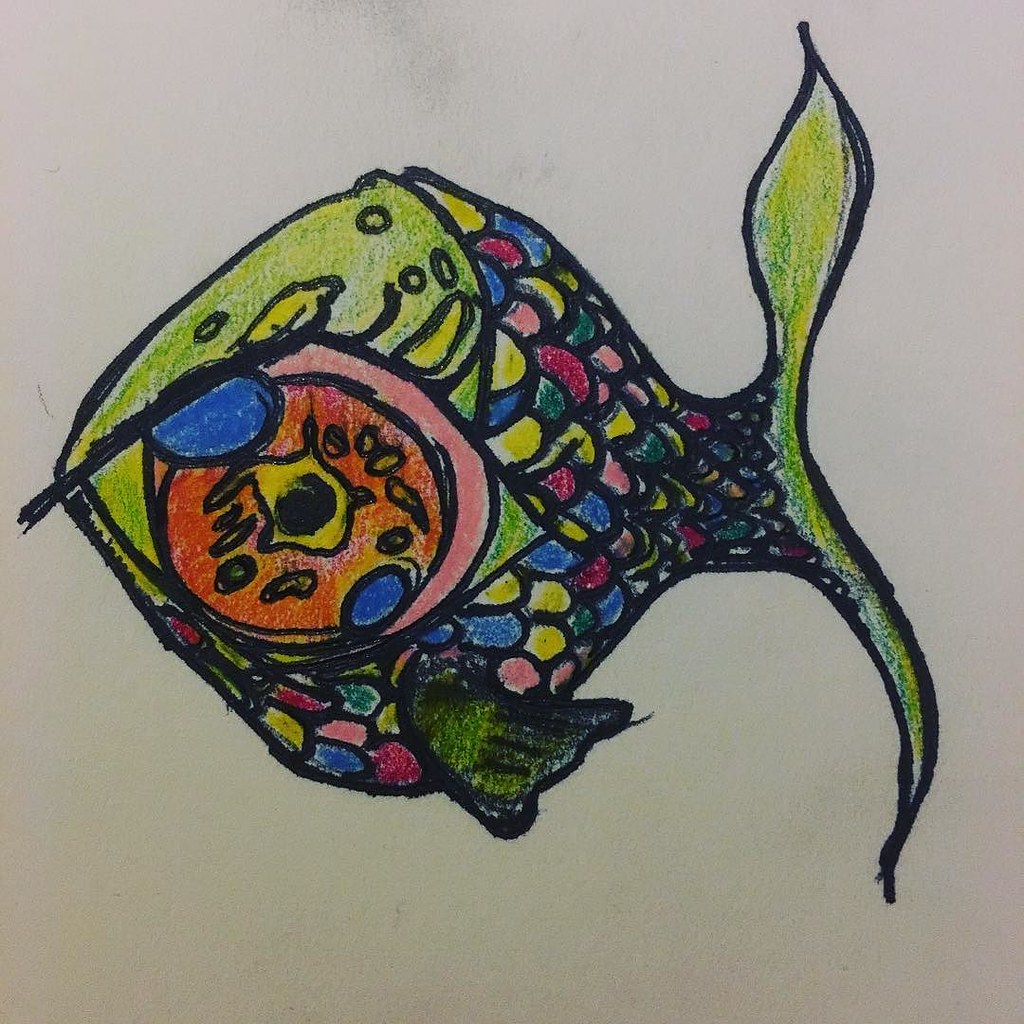This abstract-style drawing depicts a fish reminiscent of a clownfish. Set against a white paper background, the fish features a distinct shape with a tall tail that arches downward before narrowing at the body and then broadening again toward the head. The tail and the small fins on the fish's underside are vibrant green. Its body is adorned with small, U-shaped scales in an array of colors, including yellow, red, blue, and green. The front portion of the fish’s face is also green, highlighting a prominent large eye. This eye displays an intricate design, with a pink interior, two bright blue spots, and an orange circular area overlaying a yellow and black center.